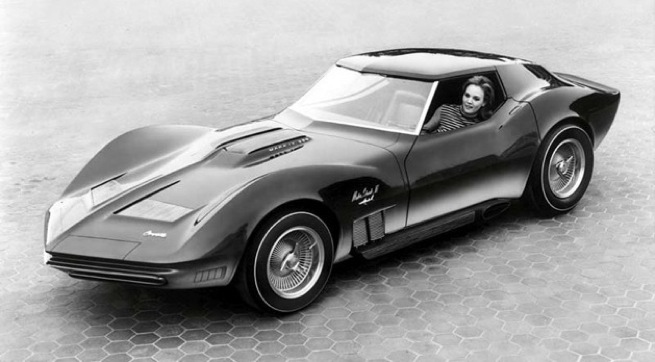A detailed black-and-white photograph captures a dark-colored, early 1970s Chevrolet Corvette Stingray elegantly parked on a geometric, honeycomb-tiled floor that stretches into the distance. The iconic sports car's rear is positioned towards the upper right of the image, while the front faces the lower left, showcasing its angular, aerodynamic body with flush headlights and striking rims. Reflective light subtly highlights the hood and the right side of the windshield. The Corvette’s recognizable logo is visible just behind the left front wheel. Seated in the driver's seat, a woman dressed in a striped top has her head slightly poking out of the window, wearing dark clothing and sporting a hairstyle reminiscent of the 60s or 70s.